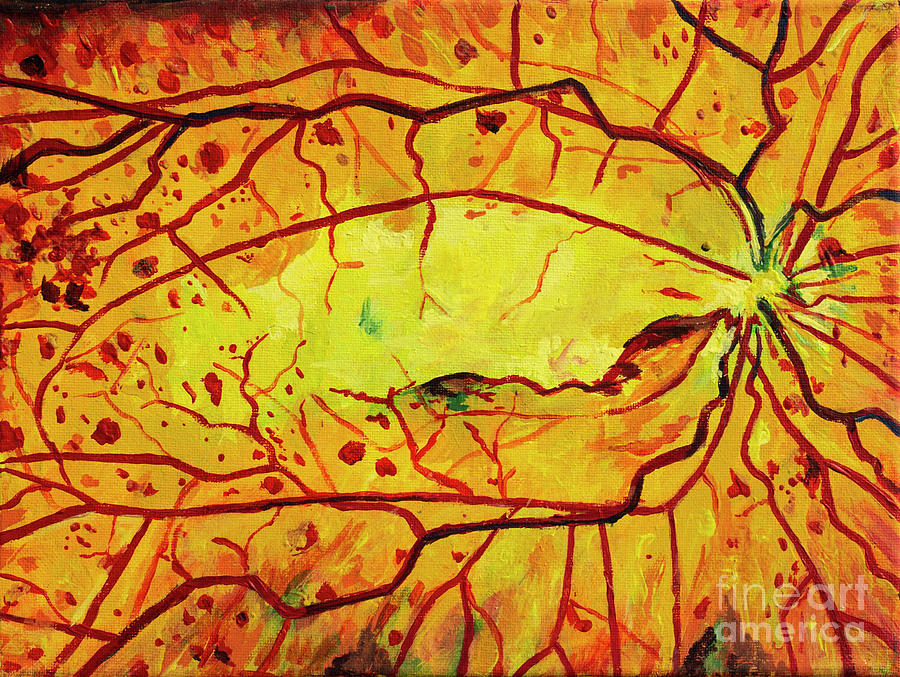The image is a captivating abstract painting that exudes a sense of luminous energy. It features a bright yellow central area that transitions into an orange middle and further into a deep red towards the edges, creating a gradient effect reminiscent of radiant sunlight or intense heat. Criss-crossing brown vines or branches dominate the artwork, originating from a focal point on the right side and spiraling outward. These lines are interspersed with red splotches along the top, bottom, and sides, adding depth and texture. Subtle hints of blue and green are visible, offering delicate contrasts. Some branches are defined with black lines, enhancing the overall depth. Additionally, the image contains text in the bottom right corner that reads "Fine Art America," grounding this vibrant piece in its artistic origins. The visible brush strokes emphasize the manual craftsmanship, enriching the painting's tactile and visual appeal.